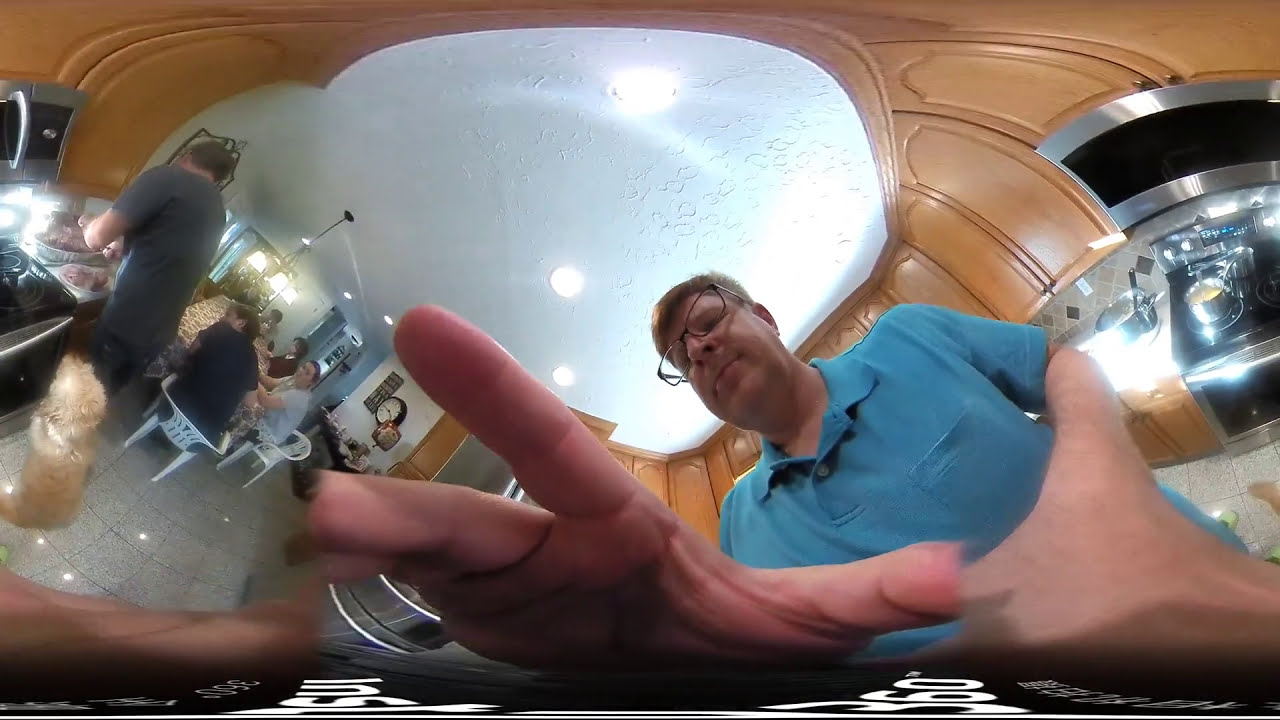The image depicts a bustling home kitchen captured with a fisheye lens, giving a curved, fishbowl-like distortion. Central to the photo is a man in his 40s or 50s, wearing glasses and a blue polo shirt. His short, grayish hair and outstretched hands suggest interaction with the camera. Behind him, the kitchen scene unfolds, featuring brown wooden cabinets, a stove, and various appliances. A brown golden retriever is positioned near another man with short brown hair, who is wearing a gray shirt and handling food in a turkey-like pan, possibly hinting at a Thanksgiving celebration. The long table, covered with a cloth, is surrounded by white plastic chairs occupied by multiple individuals, both women and men. Above the table, a chandelier with three lights hangs from a white ceiling decorated with spotlights. A clock is affixed to the white wall, enhancing the homey atmosphere further emphasized by the granite-patterned tile floor.